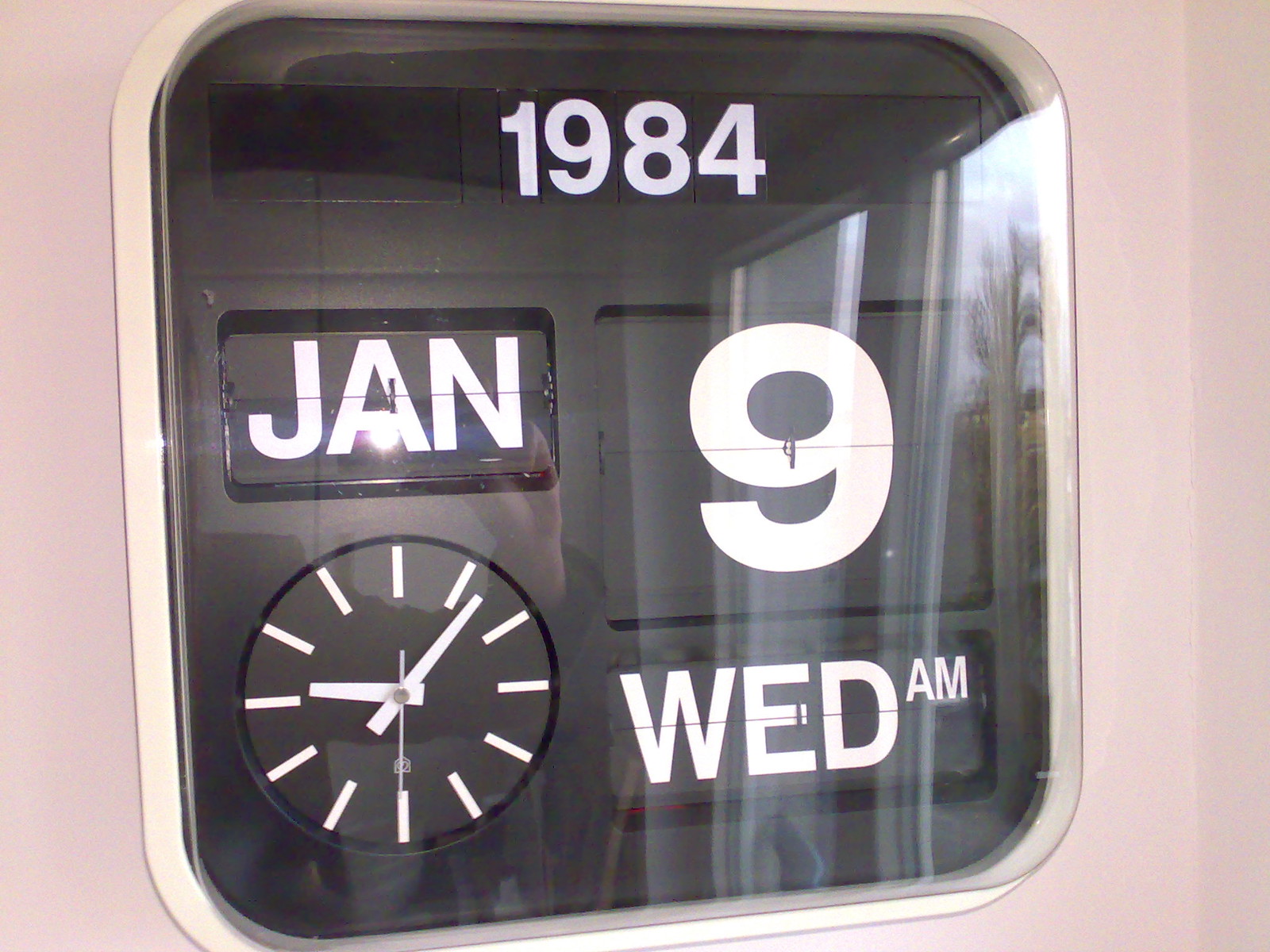This close-up photo showcases a digital clock embedded into a pale pink wall. The clock has a sleek, square design with rounded corners and features a shiny, clear plastic face that reflects the shoulder, hand, and camera flash of the person taking the photo. The clock face itself is black and segmented into multiple sections. At the top center, "1984" is displayed in white lettering, signifying the year. Adjacent sections indicate the date: "Jan" for January, and "9" for the day. There is also a round analog clock section, marked only by dashes, without numbers. The digital time reads "9:07," and another section displays "Wed. A.M.," denoting it is a Wednesday morning.